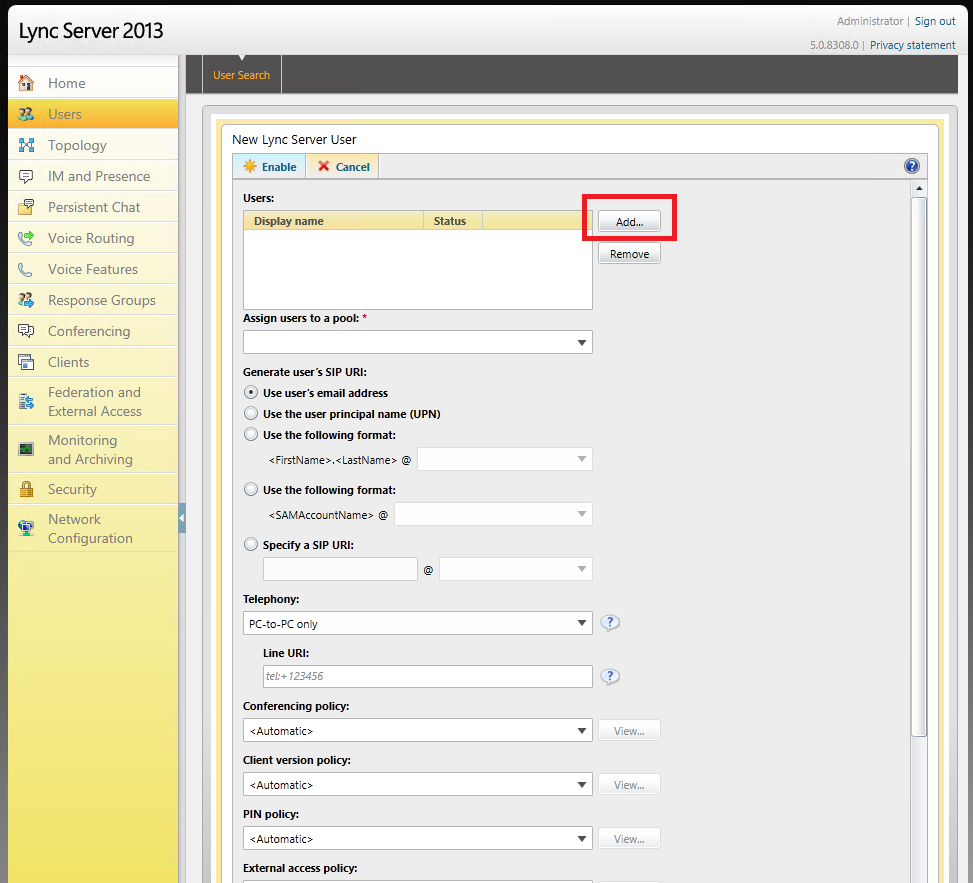The image depicts a user's workspace focused on their computer screen, presumably a work-related setting. The screen displays the interface of "Link Server 2013," indicated by the label in the top left-hand corner. Below this label, there is a vertical navigation bar with options including "Home," "Users," and "Topology," with the "Users" option currently highlighted. 

At the top of the screen, there is a "User Search" bar, featuring options to "Enable" or "Cancel." A red border highlights the "Add" button, drawing attention to it as the primary action button for adding users to the Link Server. Directly below the "Add" button, there is a "Remove" button for deleting users.

Several settings are visible in the interface, including a checkbox for using the user's email address, which is currently selected. Additionally, the "Telephony" setting is set to "PC to PC only," while the "Conferencing Policy" is configured to "Automatic."

The overall layout and highlighted elements suggest that the user is currently engaged in adding or managing users within the Link Server 2013 system.